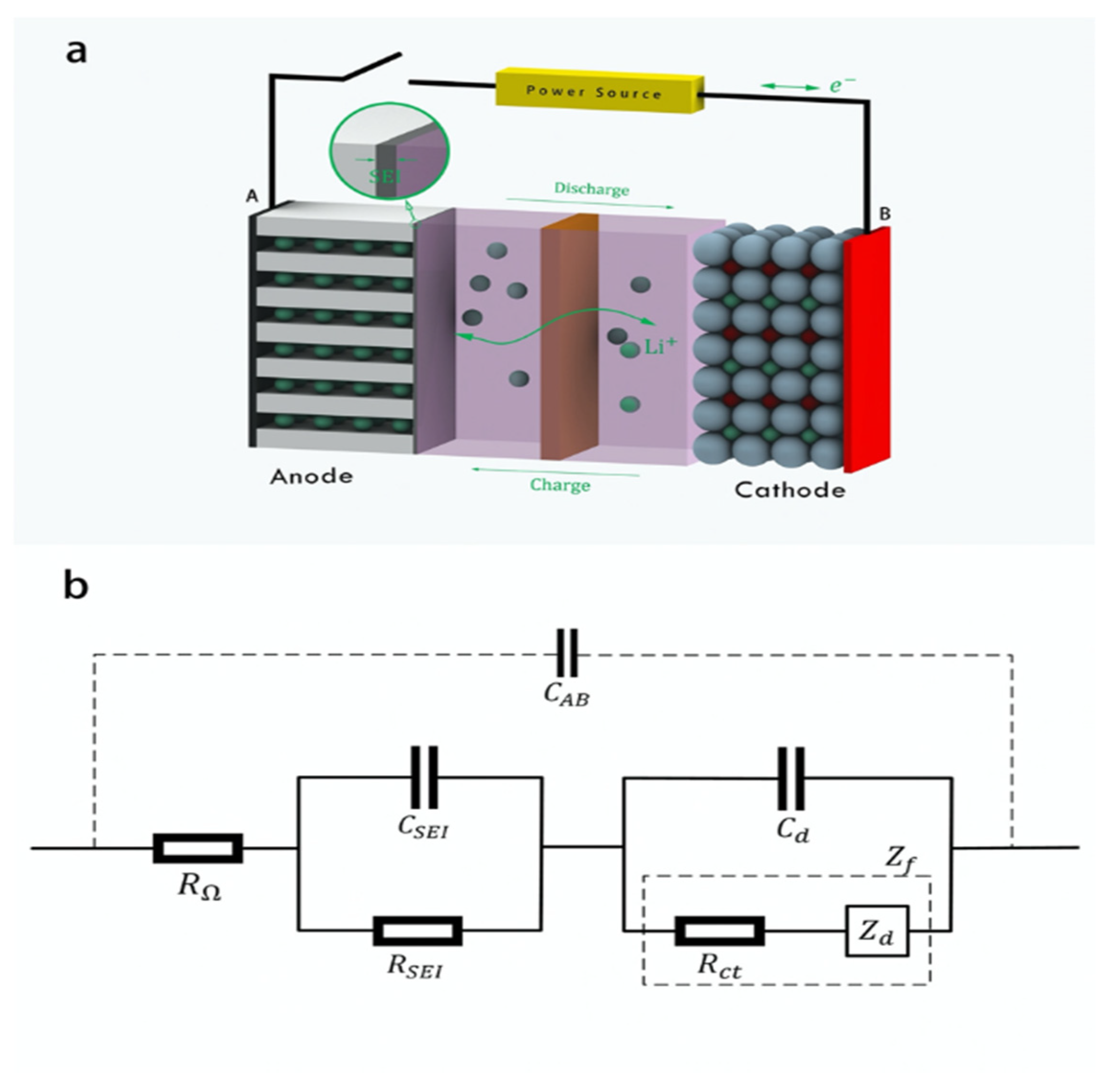The image is a diagram labeled "PowerSource," consisting of two sections: Diagram A and Diagram B. Diagram A, positioned on the upper side with a light blue background, showcases an electronic circuit involving an anode, charge/discharge mechanisms, and a cathode. The diagram includes wires, arrows, and molecules, with a color scheme of gray, lavender, and light blue, along with rectangles in yellow, red, and brown. Text annotations label various components such as anode, charge, and cathode, with the letter "A" written at the top left corner. Diagram B, located on the lower side with a white background, is a straightforward schematic featuring lines and rectangles labeled with terms like R, C set, R set, RCT, and CD. Additional components include a resistor and capacitor paralleled by a rectifier and a zener, with a larger capacitor labeled C-A-B. The letter "B" is marked at this diagram's top left corner.